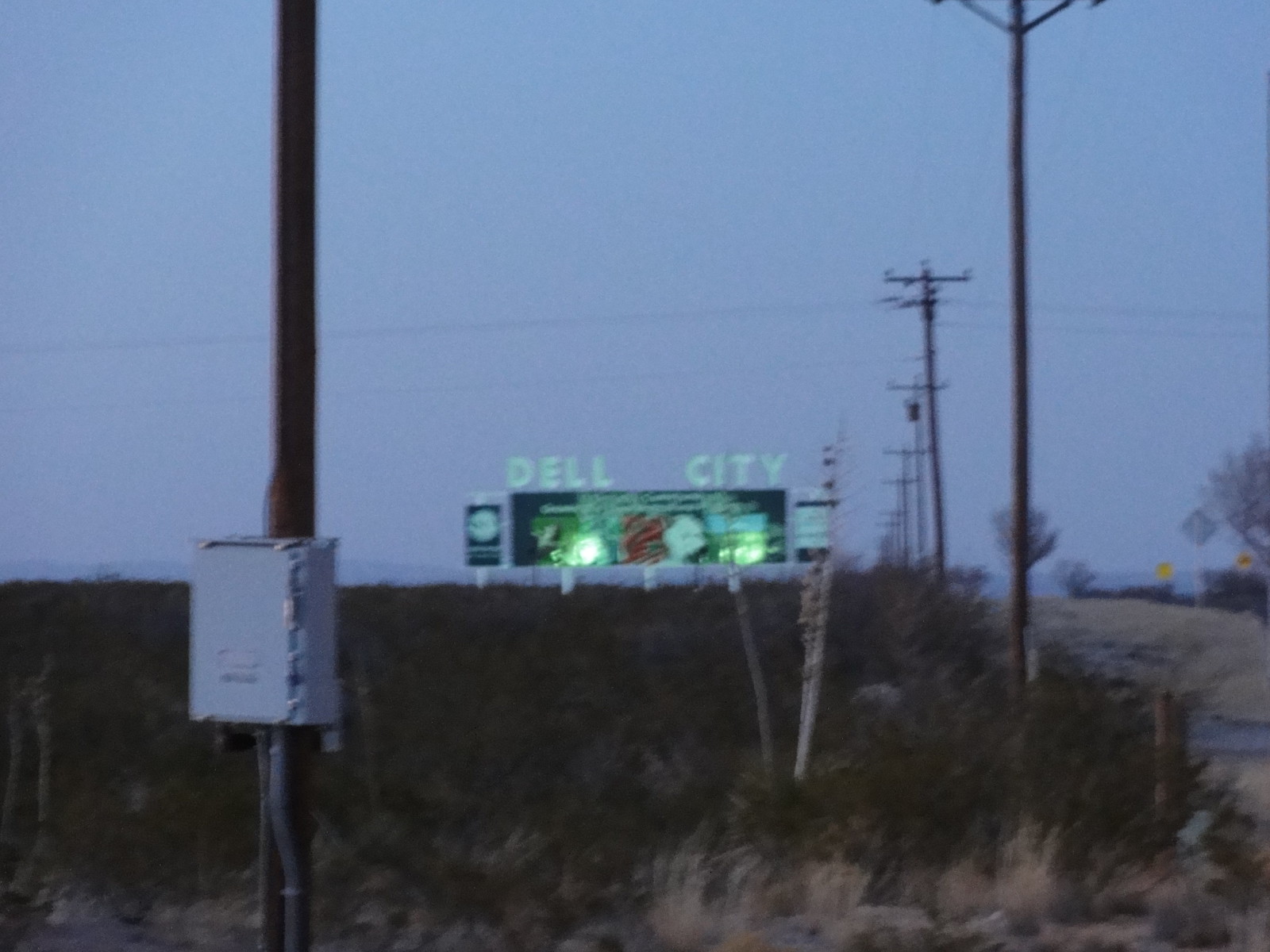A distant billboard stands against the horizon, visible across a sprawling field of untended grass and weeds. The foreground is dominated by tall yellow grasses, adding layers of texture to the image. Lining the periphery of this expanse are numerous utility poles stretching all the way to the horizon, creating a stark contrast with the natural elements. The billboard itself features a large blue banner with red and light-colored designs, illuminated by two spotlights. Above the main sign, white letters spell out "Dell City" against the open sky. Flanking this central billboard are additional signs: one blue with a white circle and some unreadable white text, and another white with blue borders, also bearing illegible writing. This scene captures a blend of human intervention and natural overgrowth, set under an expansive sky.